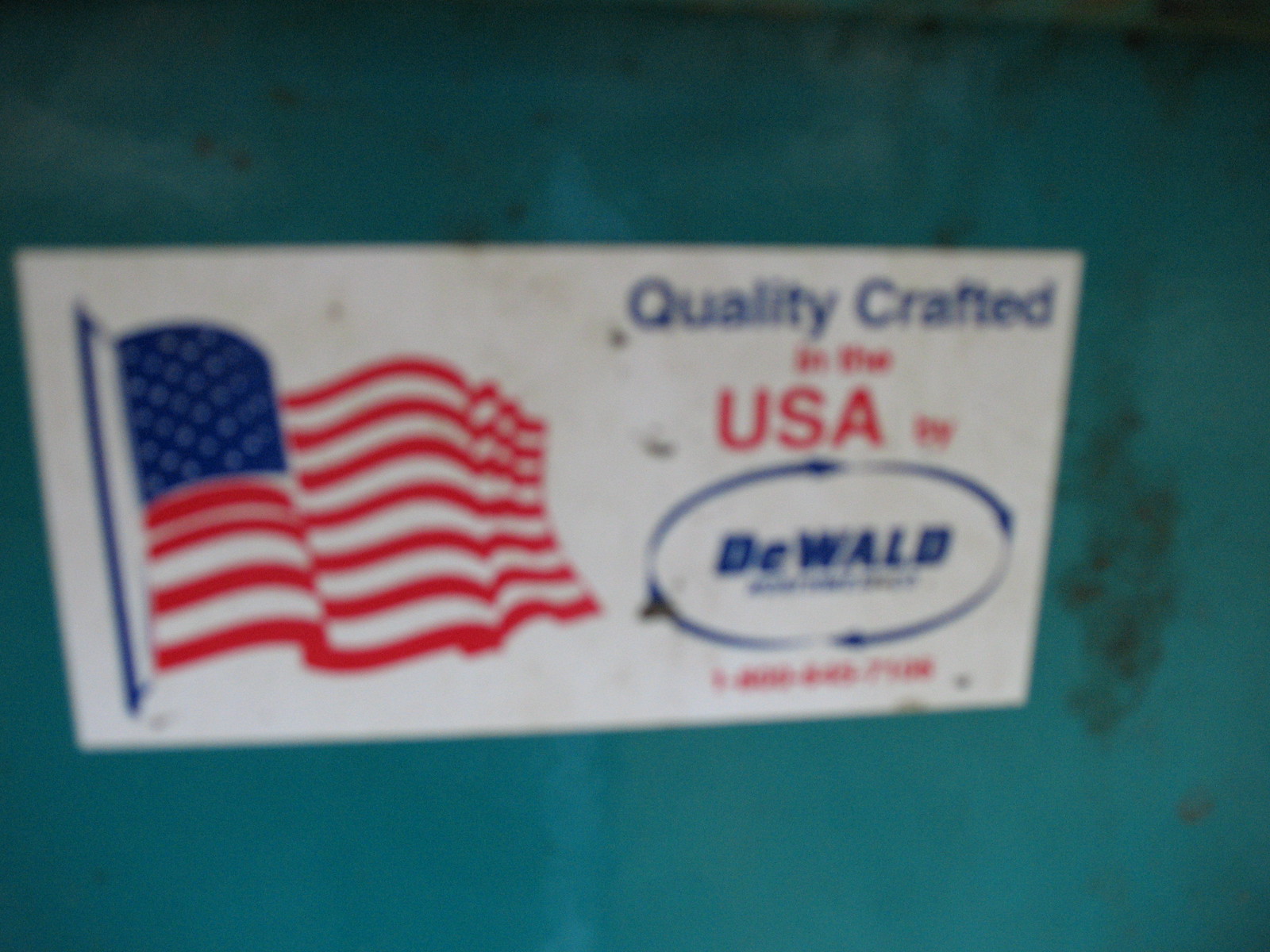A blurry photograph captures a white rectangular sticker, advertising a company. On the left side of the sticker, a waving American flag is prominently displayed. To the right of the flag, the text "Quality Crafted" appears in blue ink, followed by "in the USA" in red ink. There are small, illegible red writings next to the word "USA." Beneath this text, a blue oval contains the word "DEWALT" spelled out in white capital letters, identifying the tool brand. Below the blue oval, there seems to be a phone number written in red, although it is indecipherable due to the photo's blurriness. The sticker is affixed to a turquoise blue surface that shows signs of rust, wear, or erosion.